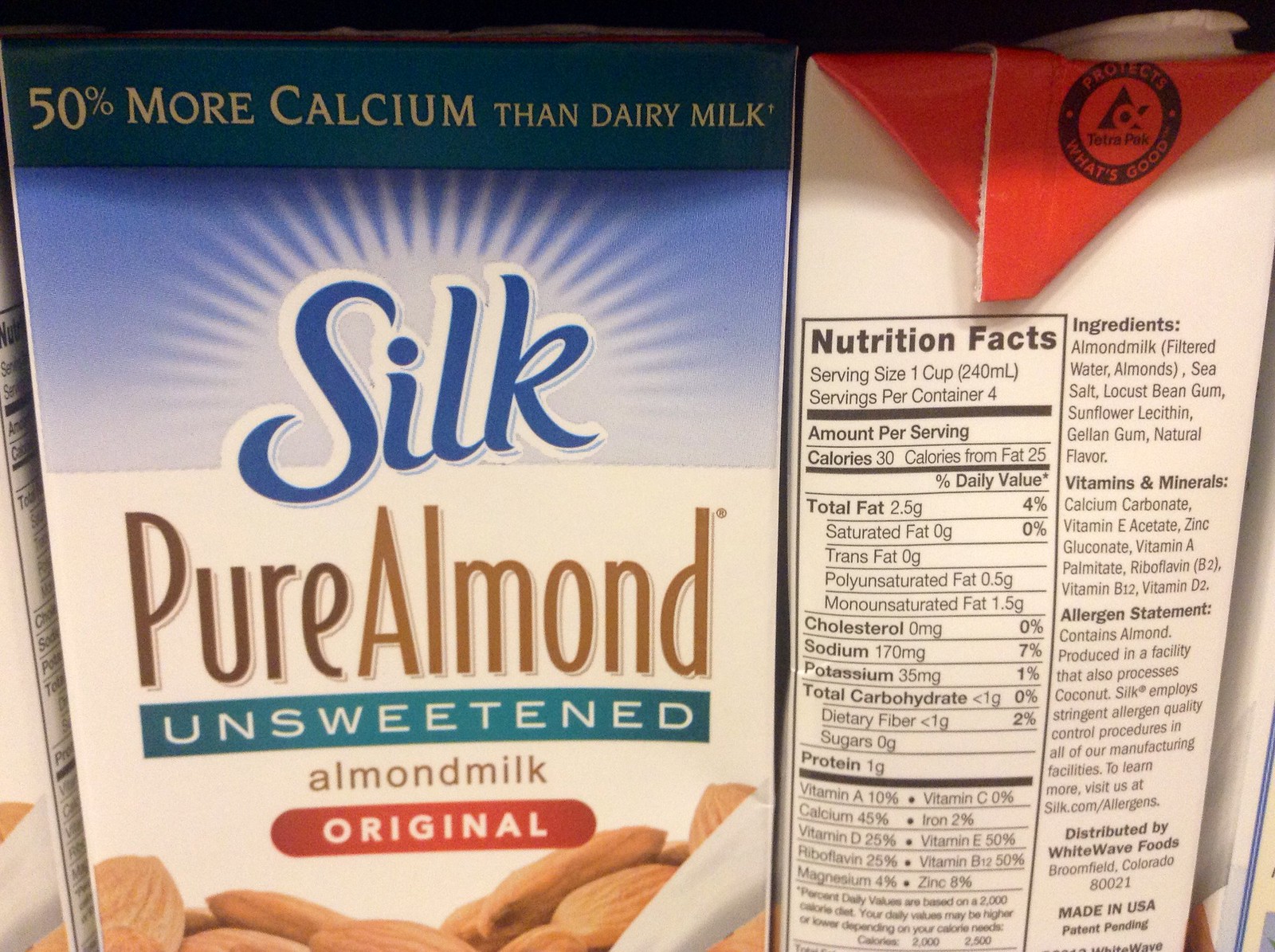A close-up image features two cartons of liquid prominently displayed. The front carton is a container of Silk Pure Almond Unsweetened Almond Milk, Original. Its design showcases a predominantly blue and white front with "Pure Almond" inscribed in brown. "Unsweetened" is written in white letters on a teal banner, situated above "Almond Milk" which is printed in a straightforward font. A vibrant red rectangle with white letters displays "Original" at the bottom of the carton. Adjacent to this, another carton is positioned side-on, revealing only its nutrition facts label and ingredients list, making it identifiable as another almond milk product. This second carton is distinguished by its red cap, indicating that it is a different variety from the Silk Pure Almond Unsweetened Almond Milk carton.